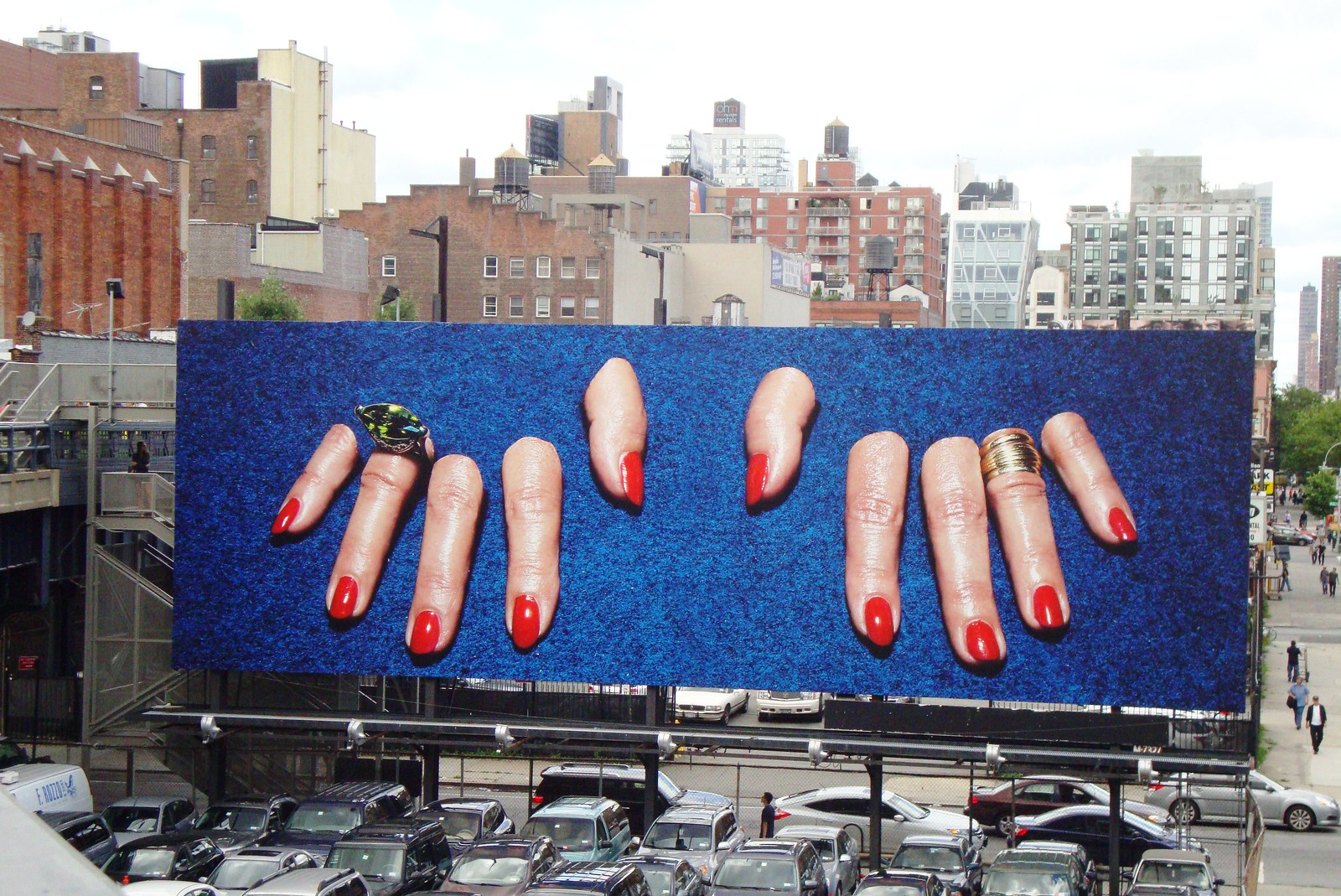In a bustling cityscape, this vivid photograph captures a large, low-to-the-ground billboard positioned just above a busy parking lot filled with numerous cars. The billboard, propped up by multiple black posts, boasts a striking dark royal blue background with a sparkly texture. The main focus of the advertisement is an array of fingers, painted with bright red nail polish, arranged to mimic the shape of hands despite the absence of visible palms. Notably, each ring finger is adorned with a ring, with the left one featuring a prominent jewel.

To the right side of the image, the scene bustles with pedestrians traversing a sidewalk and a view of trees in the background. The left side shows a stairwell with at least one visible individual, possibly ascending towards a nearby parking structure. Behind the billboard, the city continues to unfold with an assortment of buildings painted in hues of oranges, reds, light browns, and grays, all under a bright, blown-out white sky, indicating daytime. A road weaving through the city is visible, carrying a steady stream of vehicles that further adds to the urban vibrancy captured in this detailed snapshot.